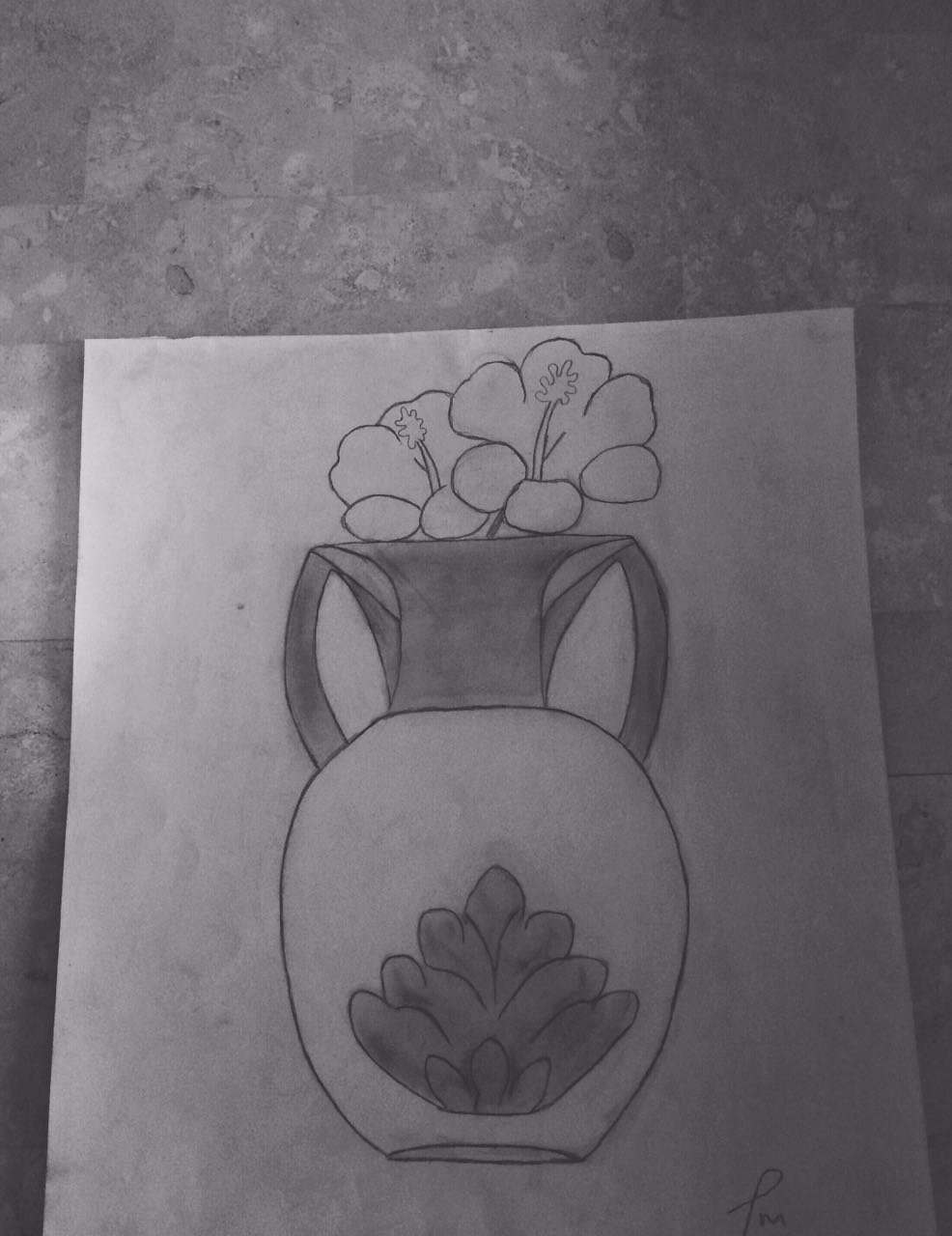A meticulously detailed pencil drawing on a piece of sketch paper is set against a gray, marble-textured surface. The paper itself is noticeably stained with pencil smudges, adding to its character. In the bottom right corner, a signature attests to the artist's identity. The focal point of the drawing is a white, round vase that narrows at the base and features two dark, gracefully curved handles and an intricately detailed neck. Emerging from the vase are two delicate flowers. Adding depth to the composition, the vase embellishes a dark brown, triangular design that splits into an intricate pattern resembling leaves or a shell.